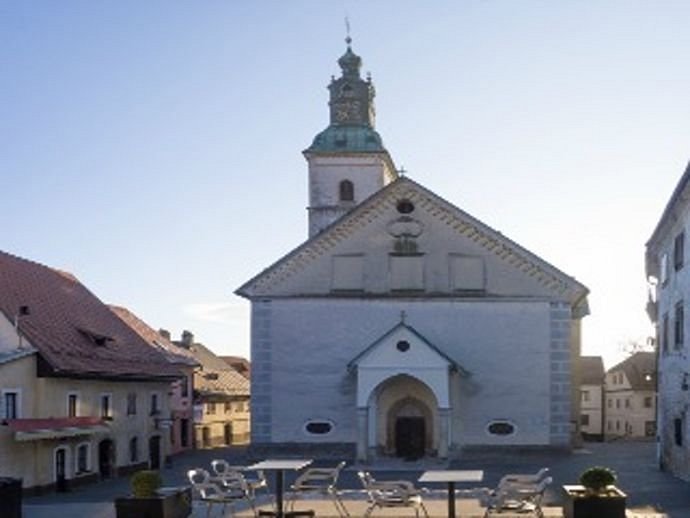This photograph captures a quaint European town square centered around a light-colored stone church with an arched entryway and a sloped, triangular roof adorned with a faint cross at the peak. Dominating the background on the left, a tall tower with a green dome and golden spire rises above the church, adding depth and historic charm to the scene. The foreground features an open courtyard with neat, rectangular tables and metal chairs, along with black potted plants, creating a welcoming outdoor seating area. Flanking the courtyard, stone buildings enclose the space: a beige two-story building with a red sloped roof on the left, and a taller, three-story building on the right. Above this picturesque setting, the horizon starts off white and blends into a pale, hazy blue sky, devoid of clouds and adding a serene ambiance to the mid-day scene. The absence of people further accentuates the tranquil and timeless atmosphere of this charming town square.